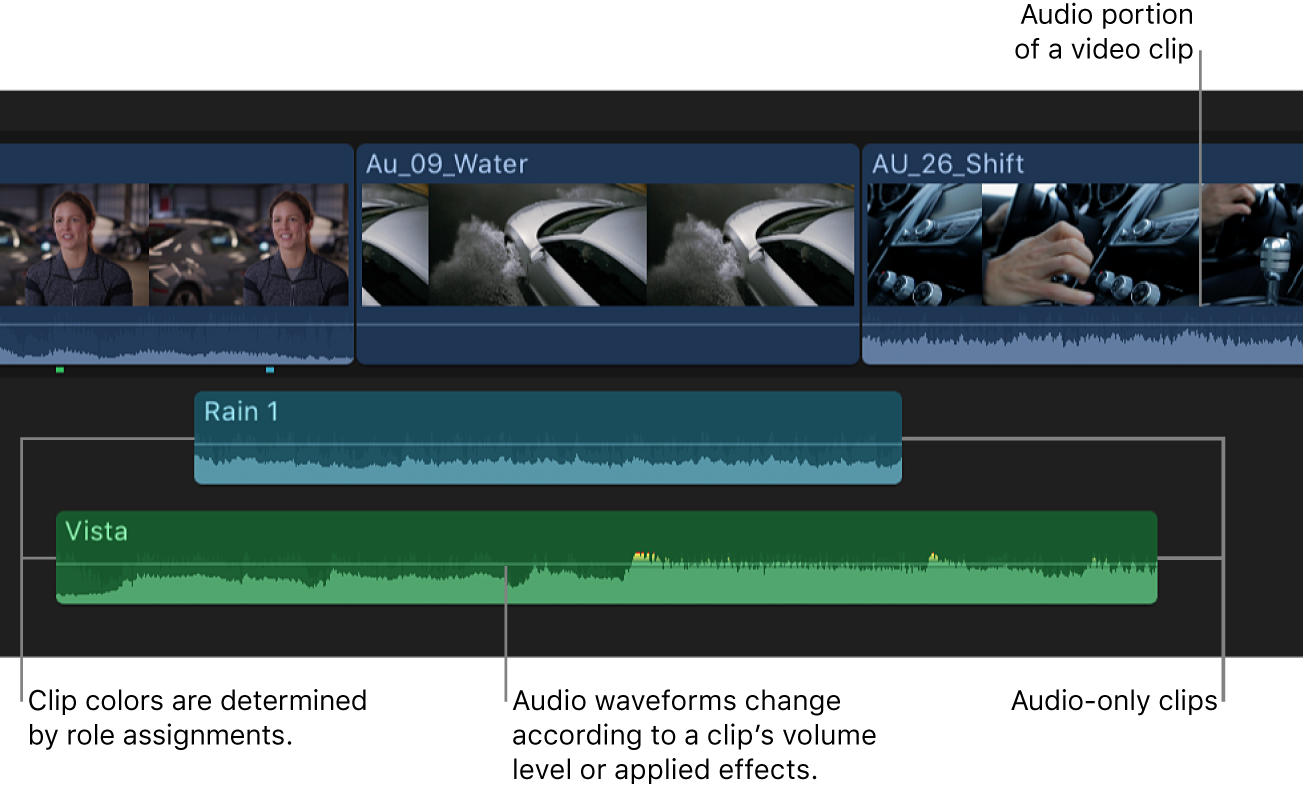The image is a detailed screenshot of an audio-video editing program, displayed on a predominantly black background. The interface features three main layers of editing: the top layer shows edited film clips, the middle layer contains audio tracks, and the bottom layer also includes audio tracks. The screenshot incorporates multiple labeled annotations pointing to various features within the program.

The labels provide specific information:
- In the upper right corner, a label reads "audio portion of a video clip" in small black font.
- On the bottom right, a label states, "clip colors are determined by role assignments."
- In the middle bottom section, a label indicates, "audio waveforms change according to a clip’s volume level or applied effects."
- Another label in the bottom right corner reads, "audio only clips."

The video clips displayed include scenes such as a woman standing in front of a car with smoke beside it, and a man's hand shifting a gear inside a car. Titles like "August 9th water" and "August 26th shift" are shown, with clips depicting a car driving through a large puddle of water. The audio sections feature notes labeled "Rain 1" and "Vista," specifically highlighting the use of sound effects and audio representation in green. The labels and lines connect the descriptive text to the respective parts of the video editing interface, providing a comprehensive overview of the program's functionalities.